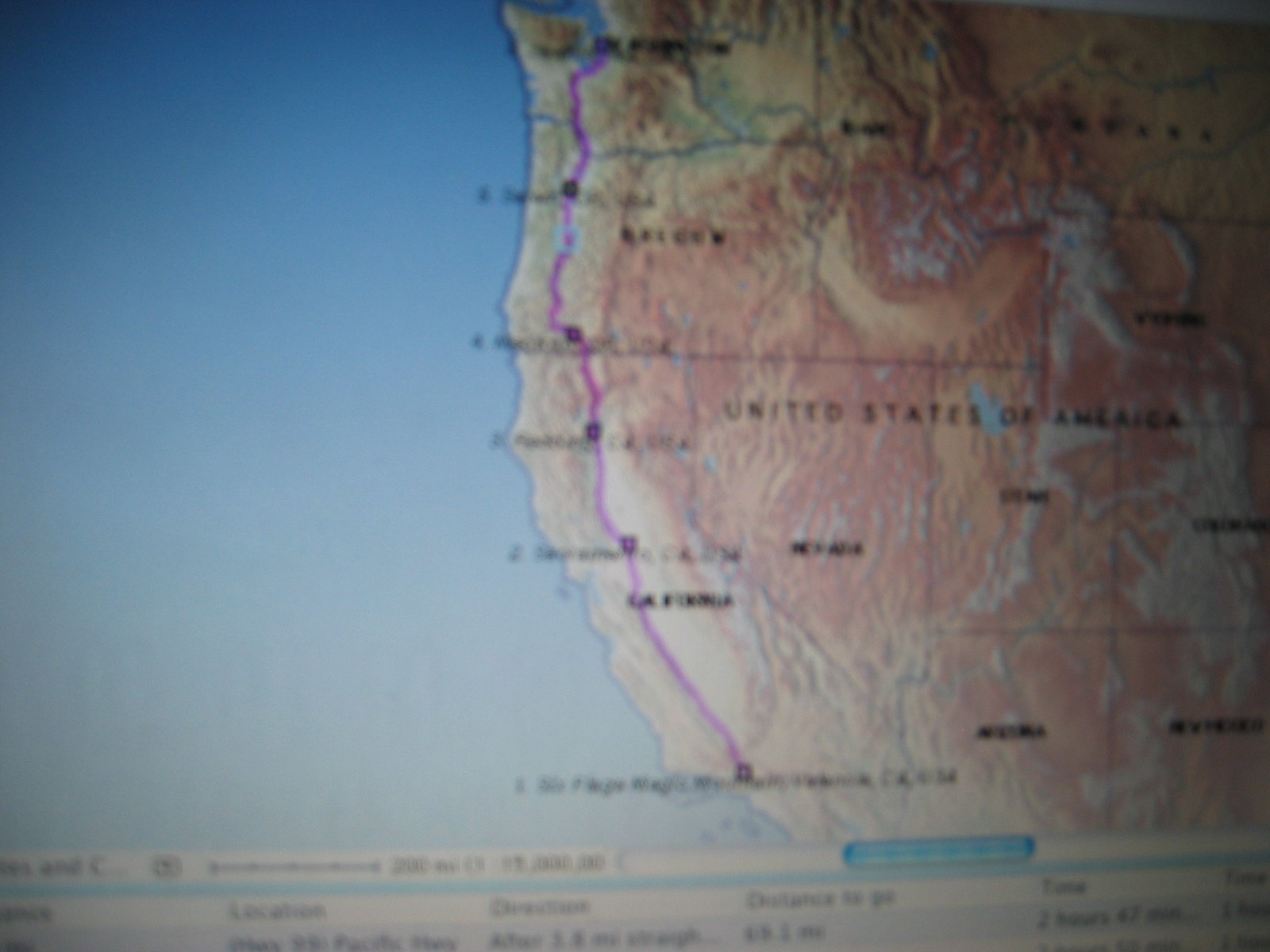This image appears to be a photograph of a highly blurred map. On the left side, it features a blue expanse indicative of the ocean. The bottom segment of the image includes a horizontal banner with a blue line, presumably meant to function as a distance scale, though the line and its calibrations are obscured by the blur. Despite this, some legible text reads "destination," "distance to go," and "time."

The right side of the image shows a brown-colored landmass, noticeably labeled with the words "United States of America" in black font, though the text is hazy. Along the western edge of this land area, there are several black dots connected by a purple line; however, the accompanying text is indecipherable due to the overall blurriness of the map.